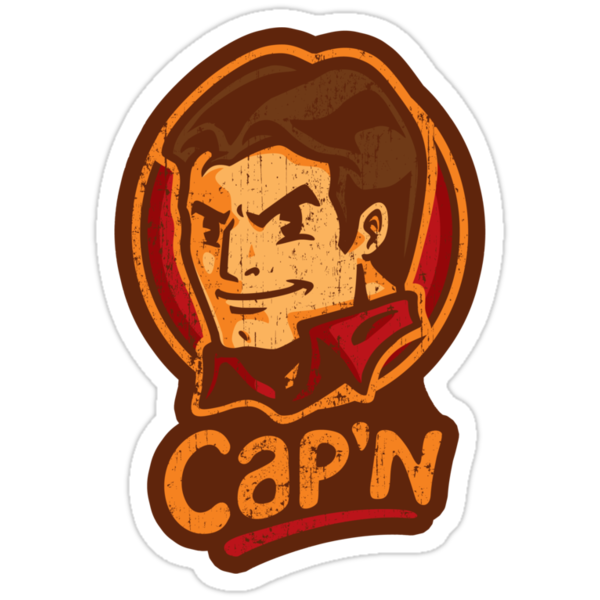This image features a sticker or magnet depicting a cartoony character named Cap'n, short for Captain. The character is a light-skinned male with wavy, dark brown hair parted down the middle, and distinctive bangs styled into a point at the front. His face is characterized by pronounced thick eyebrows that almost form a unibrow, and an exaggerated confident smile. The head and shoulders of Cap'n are shown within a circular red background framed by a yellow border that merges seamlessly into the border encircling his hair. He wears a red-collared shirt. Below his shirt collar are the words "Cap'n," written in yellow-orange text and underlined in red, against a peachy beige background. Surrounding the circular image are multiple borders: an inner dark brown border, followed by an orange border, then a white border, which adds a 3D effect due to the surrounding gray border. The white border is uniform and adheres closely to the shape of the image, reminiscent of a sticker's design. Cap'n's face is slightly turned to the left, but he looks directly at the viewer, with an overall appearance that exudes confidence and a rugged, square-jawed look.